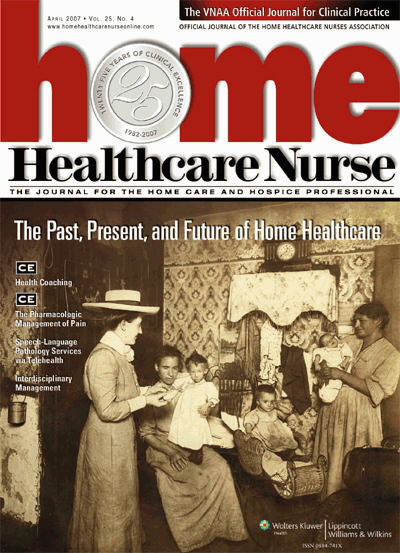The magazine cover of *Home Healthcare Nurse* from April 2007, Volume 25, Number 4, features a detailed celebration of 25 years of clinical excellence from 1982 to 2007. At the top, set against a white background with red and black lettering, the word "Home" displays a unique 'O,' replaced by a silver coin inscribed with the number 25. This coin represents the 25-year milestone of the journal. The title "Home Healthcare Nurse" is prominently displayed, followed by the official journal references and web address for home healthcare professionals.

Below the title, the cover design transitions to a sepia-toned, antique-themed photograph depicting a group of people in an old-fashioned setting. Several women, dressed in period clothing, are holding babies who are in long white gowns. Noteworthy is a woman on the left donning a large hat, adding to the historical feel of the image. This photograph sets a nostalgic tone, underscoring the theme of enduring care and the evolution of home healthcare.

Additional text over the photograph indicates the journal's focus areas, including "The Past, Present, and Future of Home Healthcare," continuing education modules on health coaching and the pharmacologic management of pain, and articles on speech-language pathology services via telehealth and interdisciplinary management. The cover also displays sponsorship logos from Walter Kluwer and Lippincott, Williams, and Wilkins, denoting industry support and partnership.

The entire cover brings together a mix of celebratory elements, historical imagery, and current professional guidance, providing a comprehensive overview for the audience dedicated to home care and hospice services.